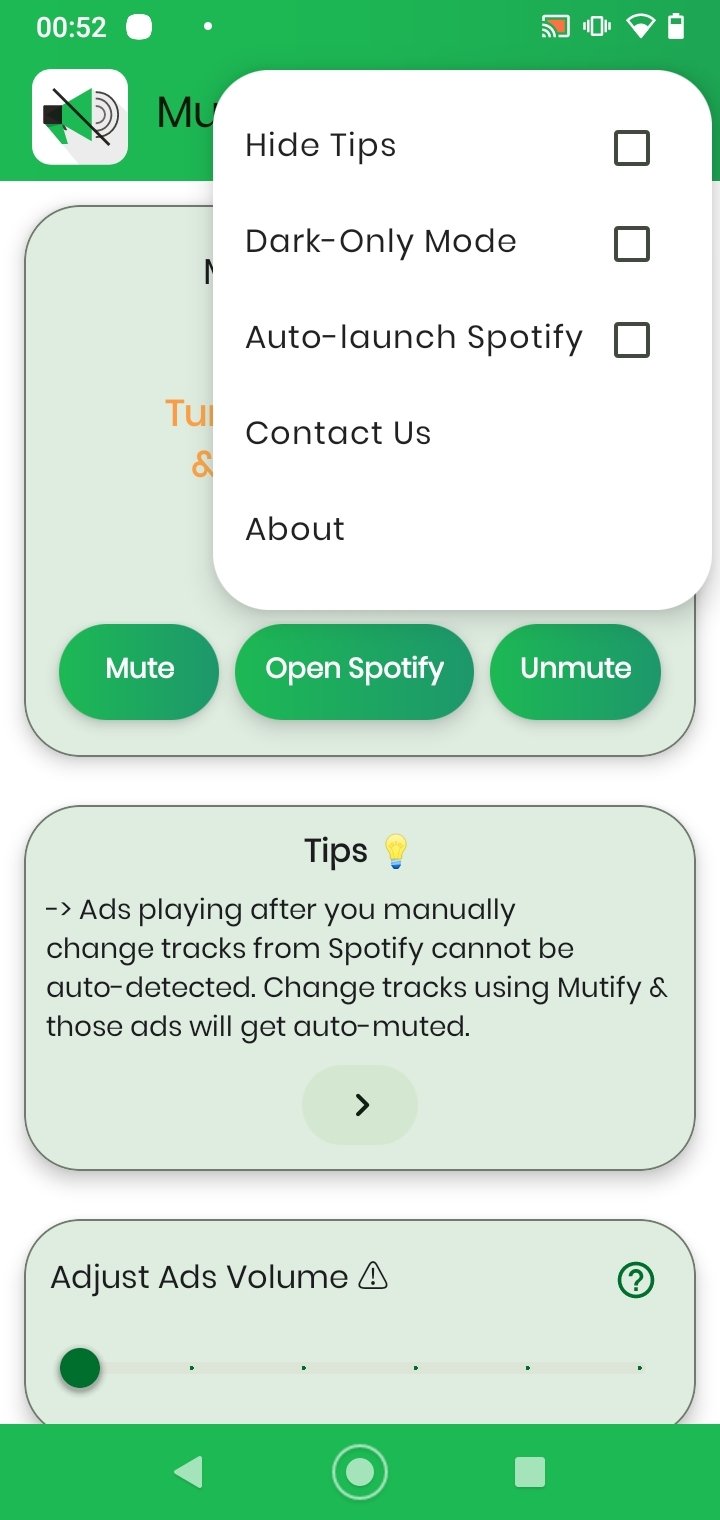The image is a screenshot taken from a smartphone. At the top of the screen, the time displayed is '00:52'. There is a green rectangle featuring a triangular-shaped icon in green, with partially visible black letters "M-U," the rest obscured by a prominent white pop-up text box. This text box contains several settings options: "hide tips," "dark-only mode," and "auto-launch Spotify," each with an associated checkbox that is left unchecked. Directly beneath these options, the text "contact us" and "about" is visible.

A pale green rectangle forms the background but is largely obscured by the white pop-up text box. Across the bottom of the screen are three green ovals labeled "mute," "open Spotify," and "unmute." Below these controls sits another pale green box labeled "tips" with a light bulb icon adjacent to it. In this box, black text explains, "Ads playing after you manually change tracks from Spotify cannot be auto-detected. Change tracks using Mutify, and those ads will get auto-muted." At the bottom of this display is another pale green oval labeled "adjust ads volume," followed by a green bar spanning the width of the screen.